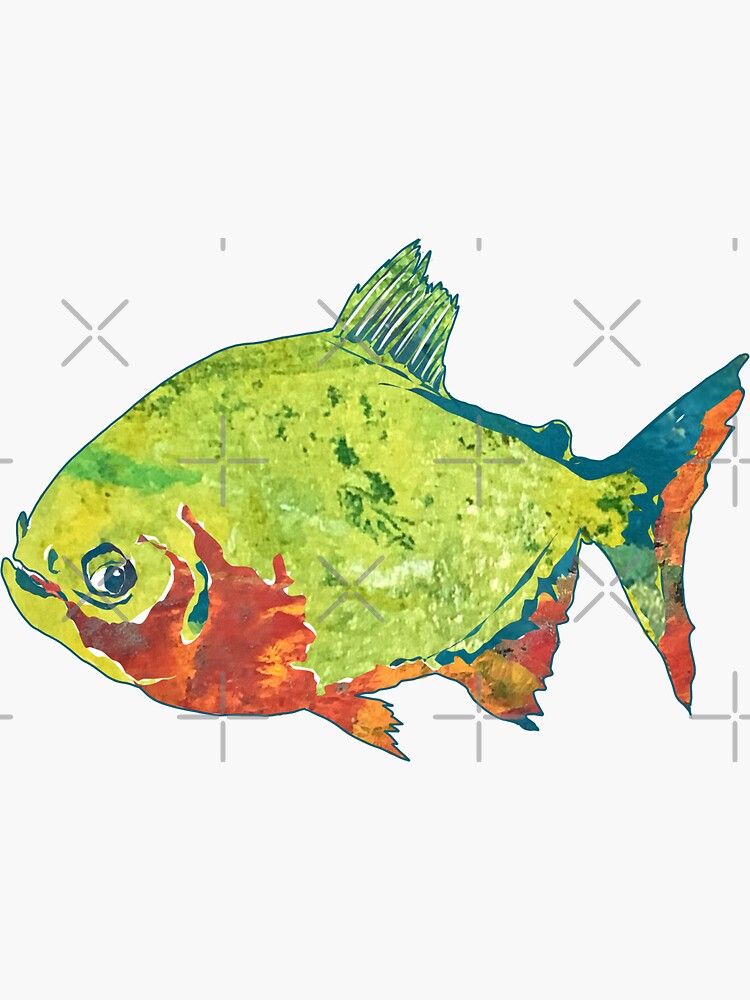This is a photo of a detailed painting featuring a piranha centered within a rectangular frame. The background is predominantly light gray, adorned with a pattern of X's and cross marks, suggesting a possible watermark or stock photo motif. The piranha, facing to the left, exhibits a vibrant color palette. Its body is an array of greens, with a notable lime green stripe near its head and aqua accents around the gills, eyes, and mouth. The underside of the fish transitions into a mix of reds, oranges, and yellows, extending to its fins and partially into its tail. The fish's eye, which bears a human-like quality, looks towards the right, while its small mouth is slightly open. The top and back fins display an aqua hue, completing the striking and intricate appearance of this aquatic artwork.